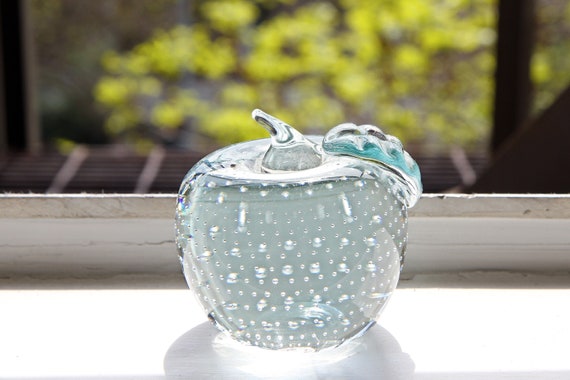In the photograph, a translucent glass apple, likely a paperweight, sits elegantly on a bright white windowsill. The apple features a delicate stem extending from the top, angled to the left, and a distinct protrusion along its right side. The glass apple, primarily transparent, creates a captivating play of light and shadow, with a white reflection and a round shadow encircling its base, cast by a bright light shining underneath it. The apple's surface is adorned with what appear to be numerous bubbles or crystalline dots, giving the impression of tiny water droplets or intricate details within the glass.

The windowsill itself is a vivid white, in front of a wooden window frame with peeling paint and casting a shadow. Visible through the unfocused window are glimpses of a vibrant outdoor scene: blurred greenery that hints at trees or bushes and bright yellow flowers. To the right side of the outdoor scene, a vertical brown bar and triangular brown shape add depth to the background. The apple also has a textured leaf seemingly crafted from blue glass, contrasting slightly with the apple's predominantly clear form. Together, these elements create a detailed and serene depiction of the glass apple resting in its bright, naturally-lit setting.